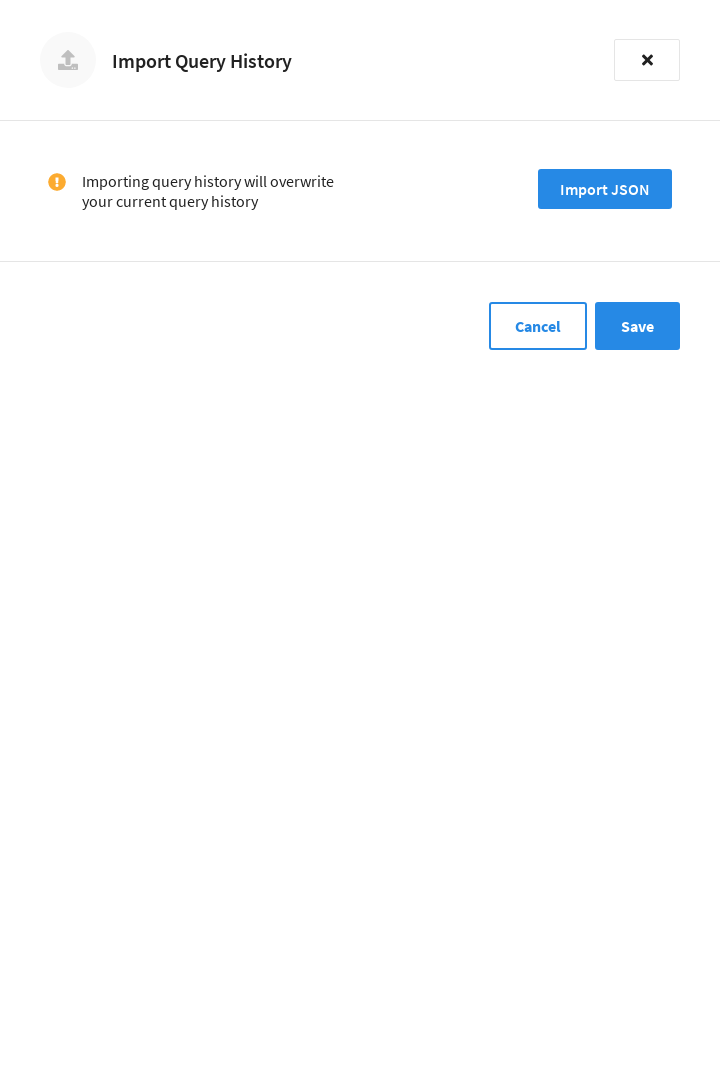This is a detailed and clean caption for the described image:

"The image shows a computer screen displaying the interface for importing query history. The background of the page is white. At the top left corner, there is a gray circle with a darker gray flat rectangle symbol inside, accompanied by an upward-pointing arrow. To the right of this symbol, the text 'Import Query History' is written in black. On the far right, there is a gray rectangle with a black 'X' inside, allowing users to exit the interface.

Below this top section, a thin gray line divides the page. On the left side of the next section, there is an orange circle with a white exclamation point. Next to it, in black text, the warning reads: 'Importing query history will overwrite your current query history.' To the right of this warning, there is a blue rectangle with white text that says, 'Import JSON.'

Another gray dividing line follows. At the bottom right corner of the interface, there are two options: A white rectangle outlined in blue with the word 'Cancel' in blue text, and next to it, a blue rectangle with the word 'Save' in white text, allowing users to save their changes."